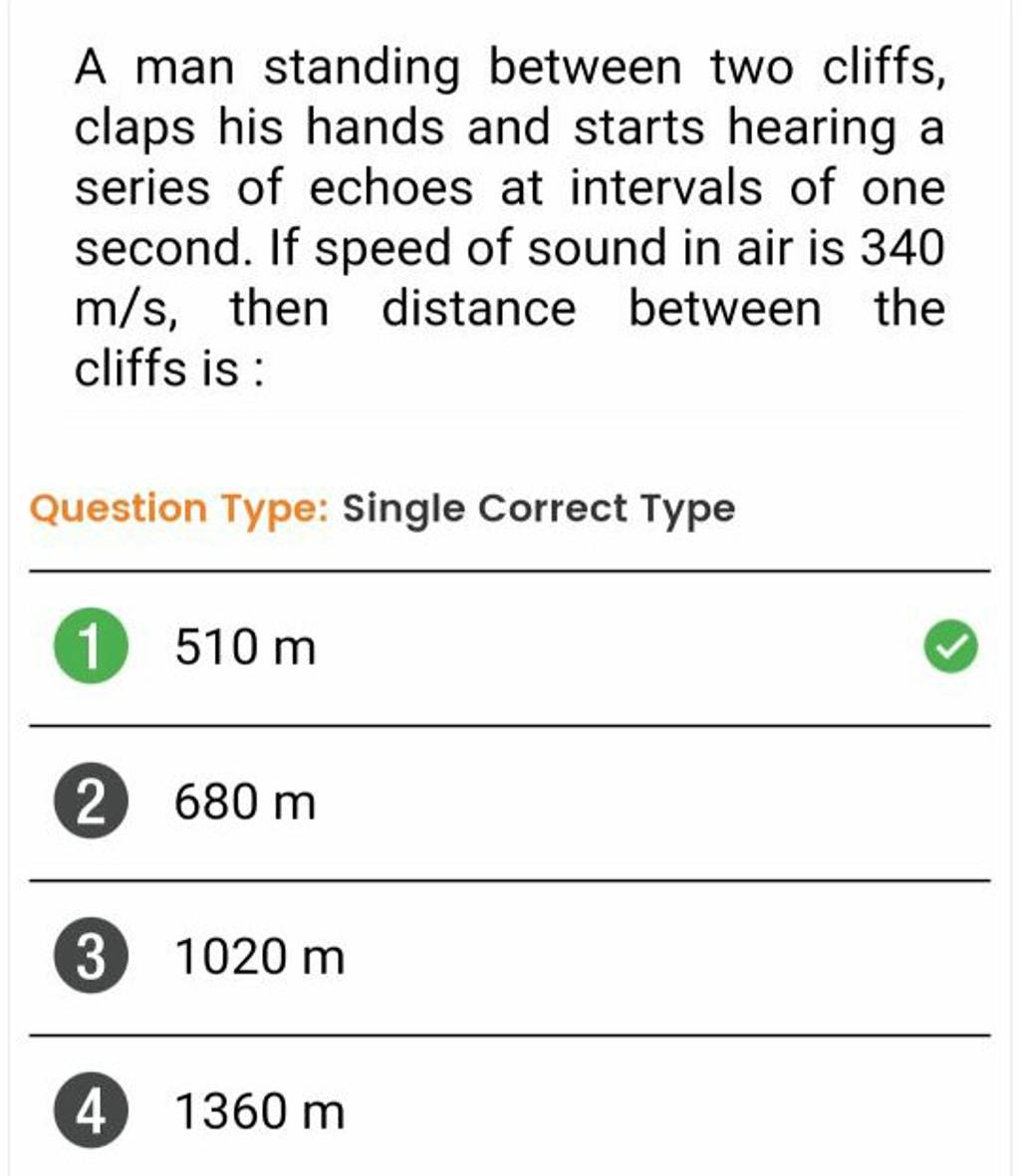The image features a screen displaying a physics problem and multiple-choice options. At the top, there is a black text that states: "A man standing between two cliffs claps his hands and starts hearing a series of echoes at intervals of one second. If the speed of sound in air is 340 m/s, then the distance between the cliffs is." Below this, in slightly blurred orange text, it reads: "Question Type." To the right, in black writing, it says: "Single Correct Type."

The screen then lists four multiple-choice options:
1. In a green dotted circle with a white "1," the first option reads "510 m" and has a green checkmark to the right, indicating the correct answer.
2. In a black bubble with a white "2," the second option reads "680 m."
3. In a bubble with a white "3," the third option reads "1020 m."
4. In a bubble with a white "4," the fourth option reads "1360 m."

The text throughout the screen is slightly larger than the standard font size typically used in text messages.